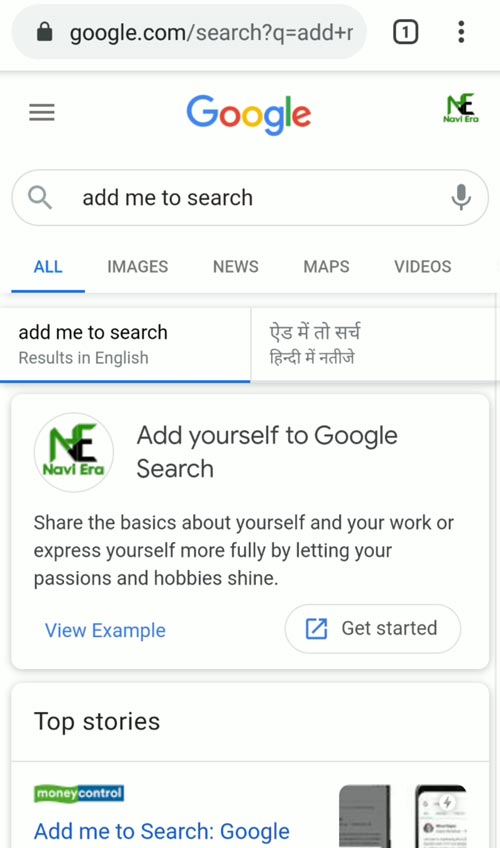A detailed and descriptive caption for the image could be:

"A screenshot of a typical Google search page is displayed. At the top of the screen, the address bar reads 'google.com/search' followed by a query. The user interface features three dots in the upper right corner and three horizontal lines on the left, next to the prominent Google logo. The search bar contains the query 'Add me to the search.' Below the search bar, there are tabs for 'All,' 'Images,' 'News,' 'Maps,' and 'Videos.' The search results are primarily in English but also include text in an unfamiliar language. The page promotes the feature 'Add yourself to Google search,' encouraging users to share basic information and their interests, with options to 'View example' and 'Get started.' A green and black stylized logo with the text 'Navi era,' which is not immediately recognizable, appears alongside top stories from 'Money Control' concerning 'Add me to search' on Google."